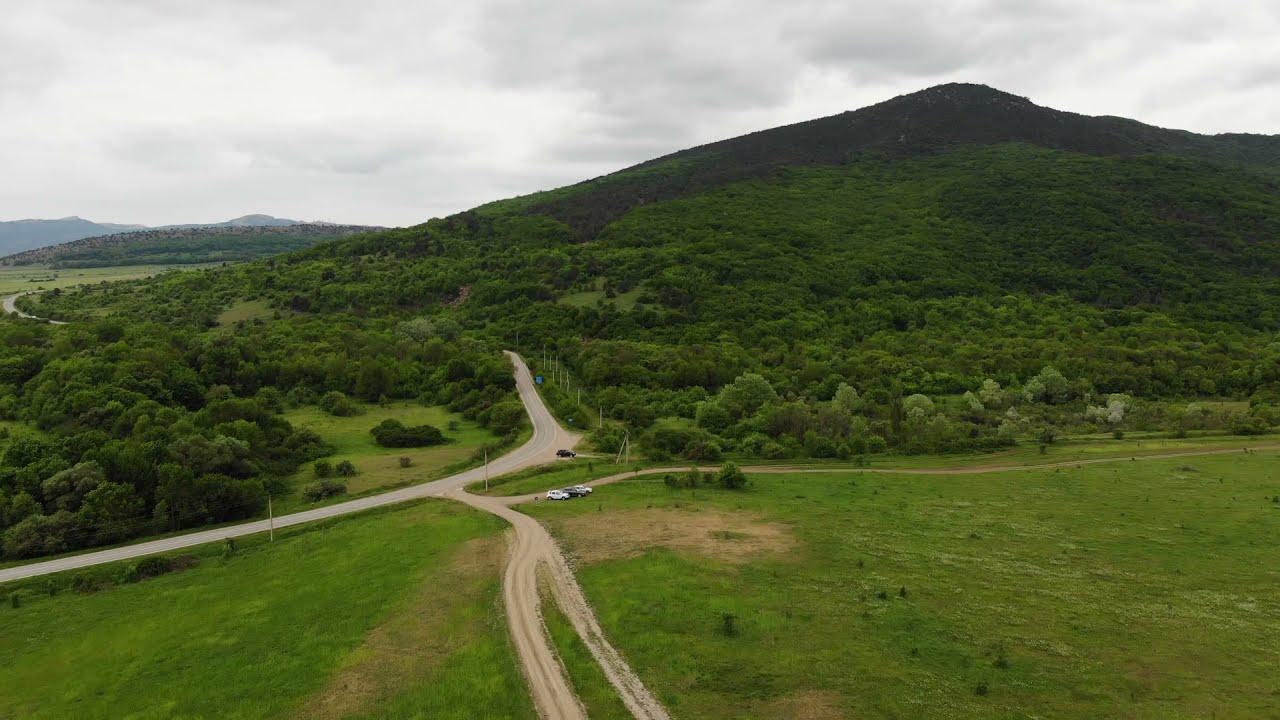This aerial photograph captures a verdant landscape dominated by three rolling hills blanketed with trees and grass. A network of roads intersects this lush scenery: a central dirt road extends upwards, flanked by grass on both sides. Diverging from this primary route, one path curves to the right while another continues straight. The straight path eventually splits into two separate roads, one transitioning into an asphalt road that arcs from the left bottom side of the image to the top left. Patches of bare earth punctuate the grassy expanse at the image's lower portion.

Near the juncture of these roads, a cluster of vehicles is visible. The middle road plays host to two white SUVs, a black SUV, and another black SUV further up the main route. The imposing hill to the center right rises dramatically, its summit swathed in clouds, reinforcing the depth and scale of this sweeping rural tableau.